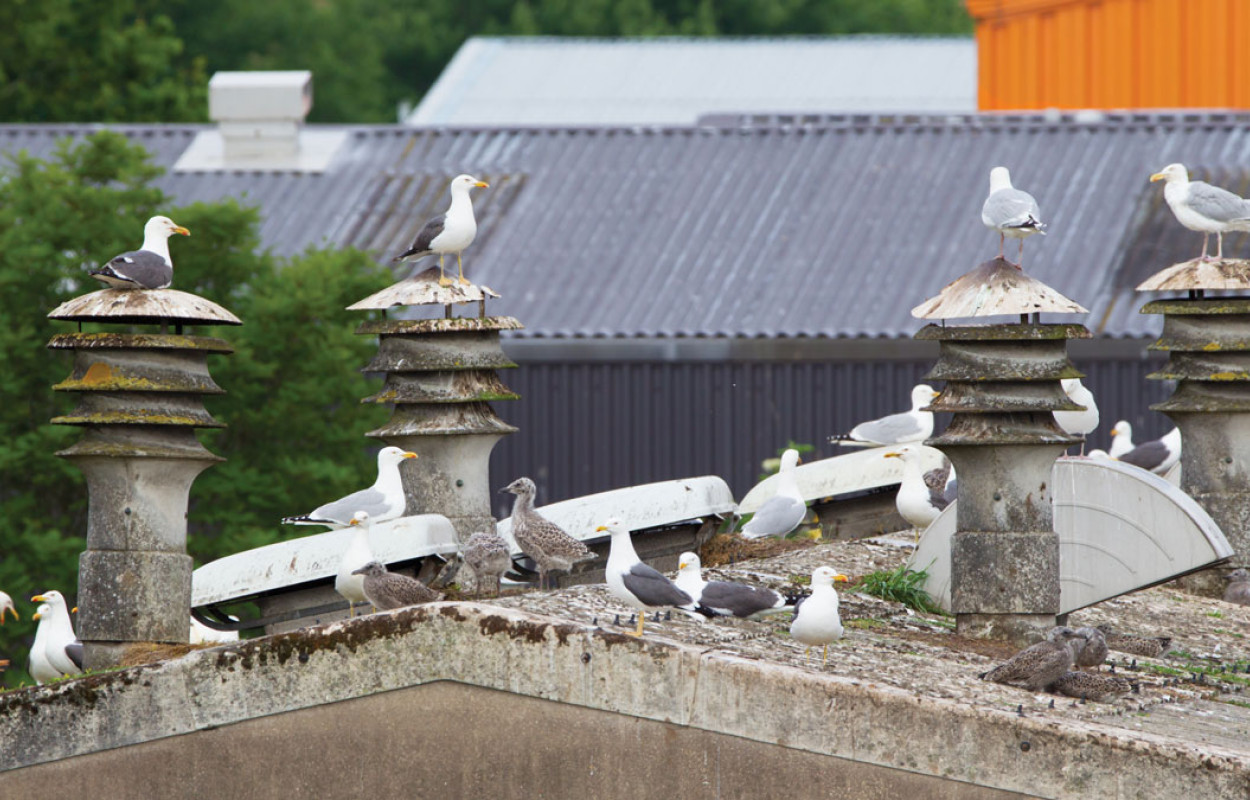This photograph, taken outdoors during the daytime, captures the rooftop of an industrial-looking building. The roof, pitched and made of whitish-gray concrete that appears aged and rusted, is heavily covered in bird droppings and some stray tufts of green grass. A notable feature of the roof is its four cylindrical metal vent pipes, each with a triangular top and a slightly rusty appearance. Additionally, there are other vents with white plastic caps scattered across the surface.

Perched all over the roof are numerous seagulls, identifiable by their white bodies, gray wings, yellow beaks, and yellow legs. Among them, a few juvenile seagulls, entirely gray, stand out. Four of these seagulls are each perched atop one of the vent pipes. Mixed among the seagulls are other birds with darker gray bodies, black beaks, and black legs.

In the background, the scene includes a treetop and several buildings with an industrial appearance. These buildings feature roofs made of corrugated metal sheets, painted in hues of bluish-gray and orange. The largest of these structures, a long and steeply pitched building made of corrugated metal, stands prominently behind the roof, adding to the industrial landscape of the photograph.